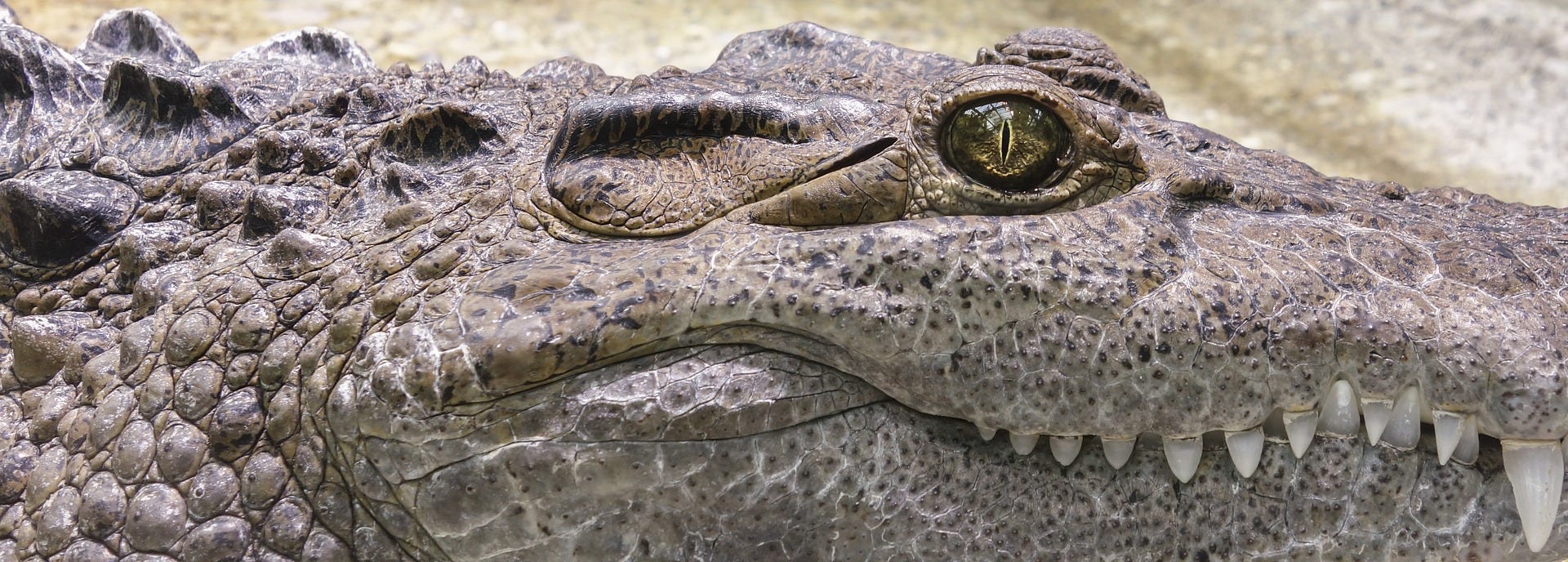This extremely close-up, side-view image captures the head and neck of a crocodile, revealing intricate details of its textured skin and predatory features. The crocodile’s eye, a rich emerald green with a diamond-shaped pupil, is prominently visible, exuding an unwavering and intense gaze directed to the right. Its skin showcases a rugged mosaic of black specks and large, unevenly sized bumps, creating a complex and tactile pattern that adds to its formidable appearance. The scaly skin coloration ranges from dark brown and tan to beige, hinting at the rough, possibly muddy environment it inhabits. The background, a blurry mix of brown and white hues, further draws focus to the crocodile's defining characteristics, particularly its sharp, white teeth protruding from the right side of its powerful jaw. Though the tip of its nose is out of frame, the image beautifully details the crocodile's head, capturing where the neck starts and the back begins to rise and curve upwards, giving a partial glimpse of its robust dorsal armor.